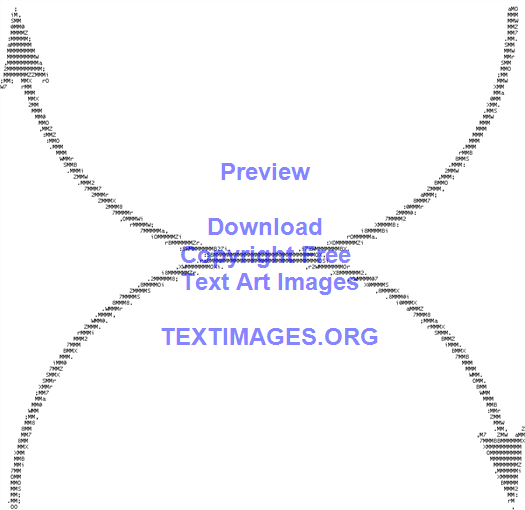The image is a digital artwork with a clean, white background, primarily featuring two intricate arrows made from a flurry of numbers, letters, and symbols, giving the artwork a pixelated effect. One arrow curves upwards to the left, while the other curves downwards to the right; they touch at the middle, forming a visually compelling design. These arrows are colored in gray or black, contrasting sharply against the white background. In the center of the image, there is purple-hued text that reads: "PREVIEW DOWNLOAD COPYRIGHT FREE TEXT ART IMAGES." Beneath this text, in all capital letters, it says "TEXTIMAGES.ORG."